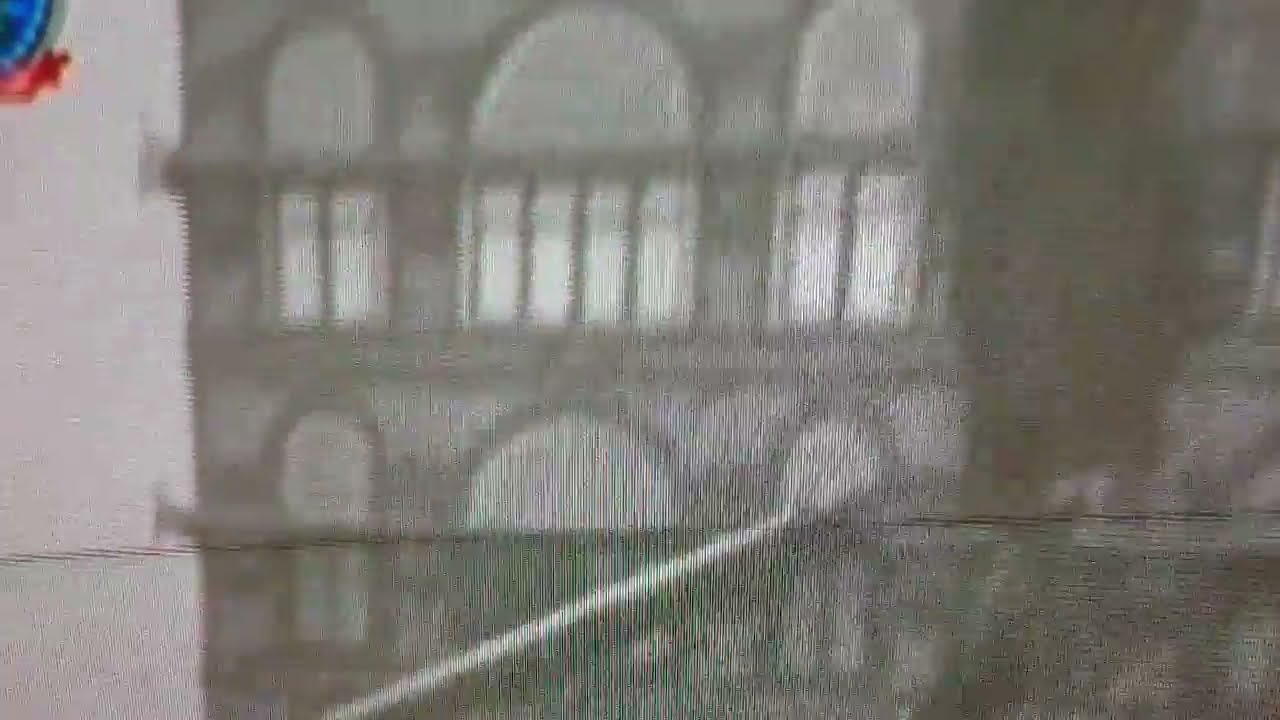This image depicts a highly vague and out-of-focus representation of a building. The building, which seems to be captured as a shadow or through a painting or drawing, is characterized by its two levels, each featuring large arched windows—three windows per level. The upper level includes a banister or balcony railing in front of the windows. The overall color scheme of the image is dominated by varying shades of grey, with lighter and darker areas contributing to the indistinct and blurry quality. On the right side, the image becomes even more obscured, with a darker grey swath descending from the top to the middle, fading further details. In the lower right, the lack of definition continues with an indistinguishable darker area. The building or its shadow appears to be slightly reflected in the lower part of the image. Notably, in the upper left corner, there is a small splash of color, showing a tiny bit of blue and red amidst the monochromatic hues. This touch of color, possibly resembling a ribbon or splatter, stands out against the otherwise grey and white backdrop.